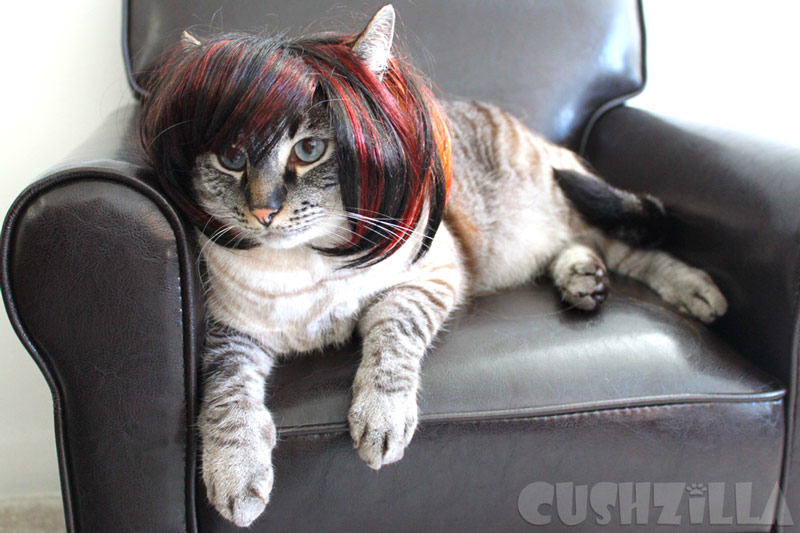In this whimsical photograph, a typical gray, white, and brown-striped tabby cat lounges comfortably in a miniature, black-faux leather chair, custom-made to fit its size. The cat's light blue-greenish eyes gaze forward and slightly to the left, its little pink triangle nose peeking out beneath a striking layered bob-style wig. The wig, vividly colored in black with red and orange stripes, features short bangs that rest just above the cat's eyes. The feline is stretched out on its stomach, with its front paws and little toes draped over the front edge of the cushioned chair, while its back legs rest towards the left side. The background is primarily white, framing the amusing scene. At the bottom-right corner of the photograph, bold text reads "Cushzilla," with the 'i' cleverly dotted with a paw print, perhaps hinting at the brand or product being showcased.